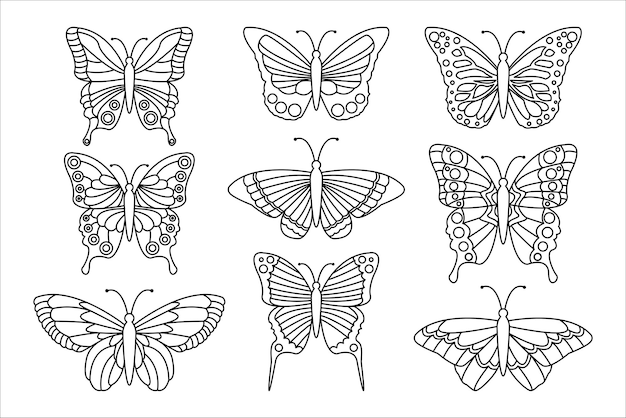This is a black and white landscape illustration featuring nine unique butterflies, which could possibly include some moths. The layout consists of three rows and three columns, positioning the butterflies evenly across the page. Each insect is depicted with its wings outspread and showcases distinct patterns - some adorned with circles, others with lines. Though the designs vary in intricacy, they maintain a relatively simple and consistent pencil sketch style with black outlines. The background remains completely white, making it resemble a page from a coloring book. Every butterfly has a pair of antennae extending from their heads, and their different wing shapes and patterns invite individual customization.